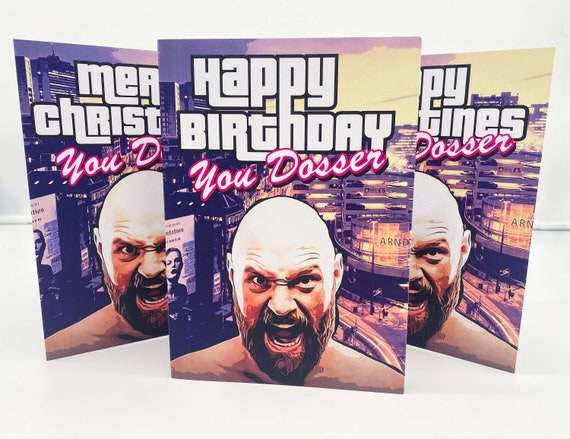The image features a series of three rectangular cards arranged in a triangular formation, each standing with a gray background. The cards prominently display an angry, shirtless bald man with a mustache and beard, whose ferocious expression reveals his teeth. The man is set against a backdrop of a purple-shaded cityscape that appears to be viewed from high above. Each card bears a different greeting at the top in white text, outlined in pink. The foremost card reads, "Happy Birthday, You Dosser," while the left card likely says, "Merry Christmas, You Dosser." The right card is partially obscured but is assumed to read something similar, possibly "Happy Valentine's, You Dosser." The style of the text has a strong resemblance to the font used in Grand Theft Auto game titles, suggesting a possible inspiration from the video game.